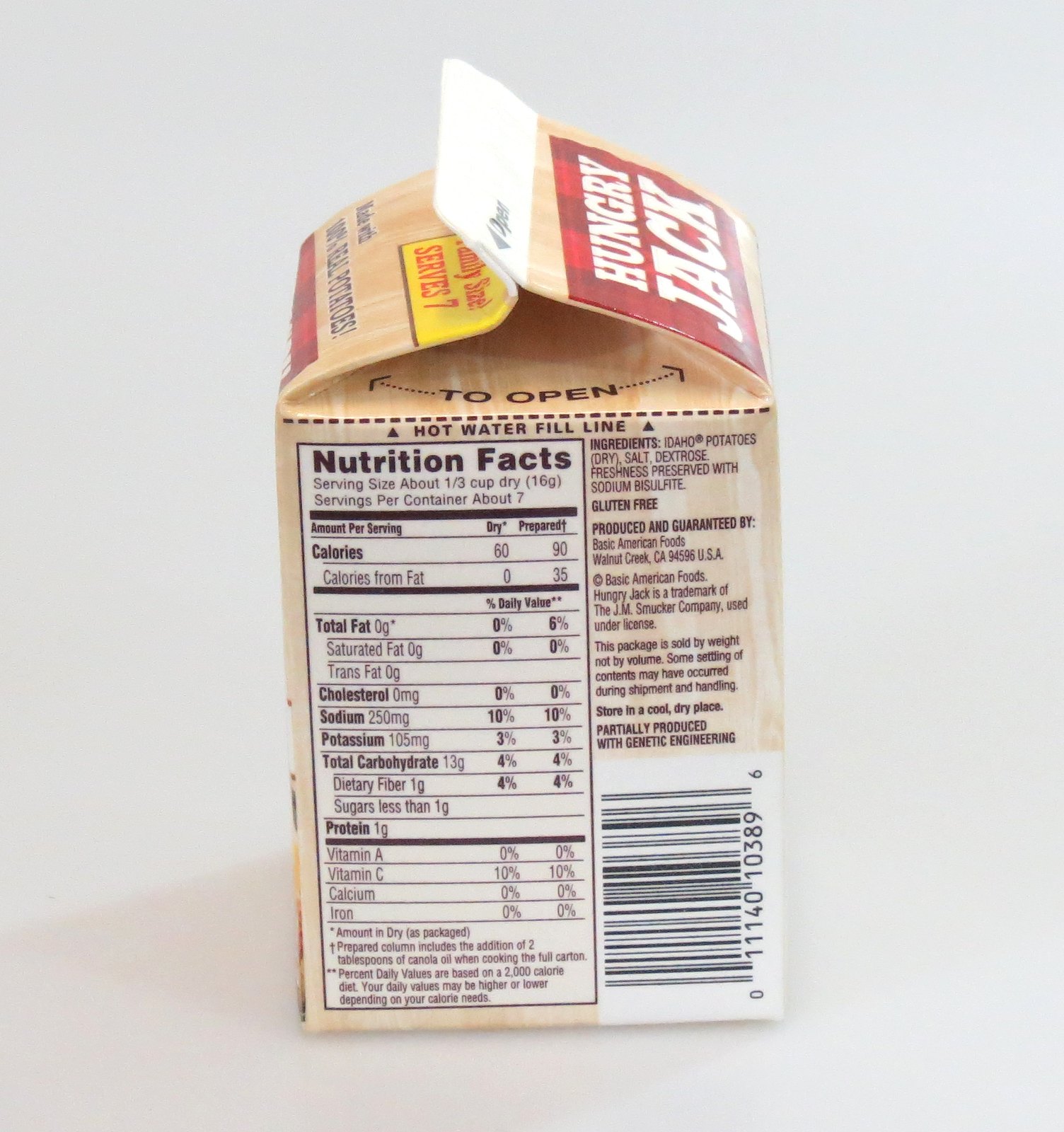The photograph captures a square, brown carton with a triangular top, prominently featuring the brand "Hungry Jack" in white lettering on a red sticker located at the top right. A checkered dark red pattern adorns this section, adding visual interest. The carton contains a detailed nutrition facts table on its left side, listing ingredients such as Idaho potatoes (dry), salt, dextrose, and sodium bisulfite, ensuring freshness. It emphasizes that the product is gluten-free and produced by Basic American Foods in California. The carton is labeled as "family size," capable of serving seven people. Instructions for opening, which include the phrases "to open, squeeze and pull apart" and "hot water line," are noted on the top, and the bottom right corner of the carton displays a barcode. The carton rests on a white surface, illustrating a functional, convenient packaging for quick preparation of mashed potatoes suitable for small to medium gatherings.